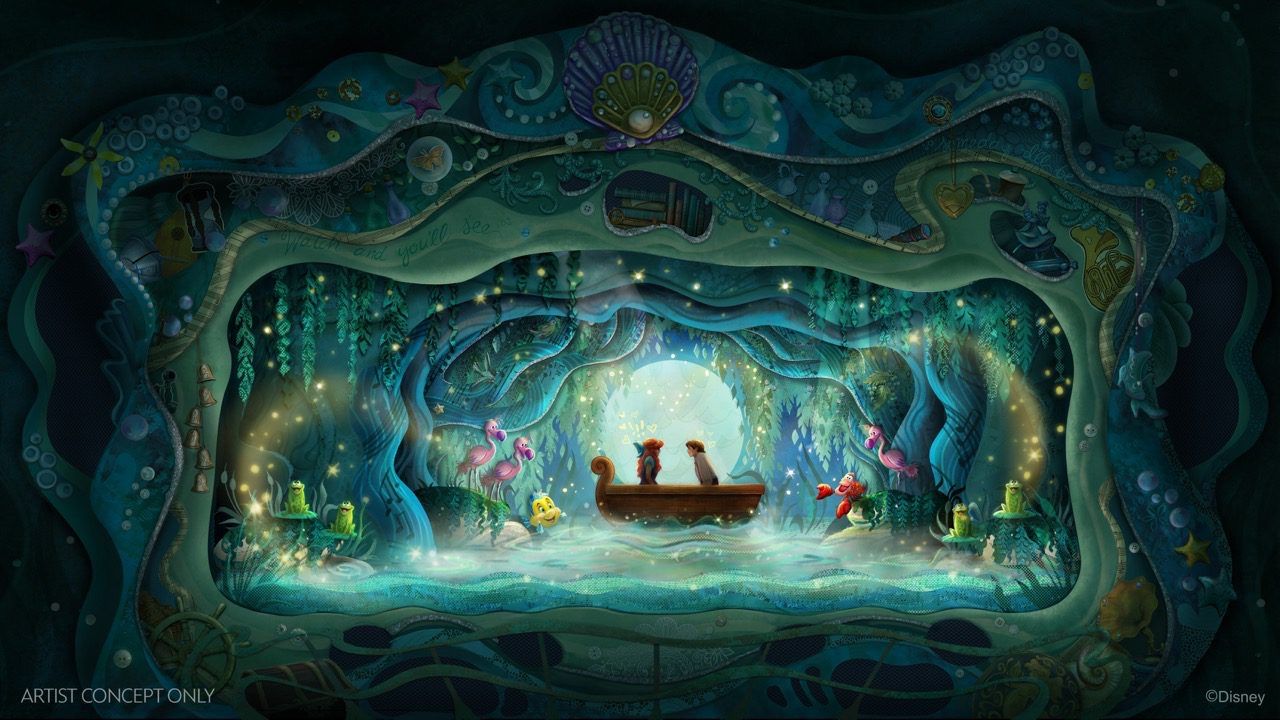The image is a highly detailed, surrealistic depiction of an underwater fantasy world, reminiscent of a scene from "The Little Mermaid." The central focus is on a brown boat with two people inside, gazing at each other. Behind them, a luminous, circular light creates an impression of entering another realm. The surrounding underwater cave is filled with blue, green, and turquoise hues, adorned with intricate sea-themed elements.

The environment is vibrant, featuring playful interactions among various creatures. Several pink flamingos, frogs on lily pads, a smiling yellow character (perhaps a clownfish), and a red lobster populate the scene. Additionally, a round portal hints at magical transitions between different worlds. The border of the image is richly decorated with seashells, seaweed, flowers, ferns, and other nautical artifacts, contributing to the overall mystical atmosphere.

In the left corner, text reads "artist concept only," suggesting an imaginative, almost magical quality to the artwork. This intricate frame further enhances the underwater theme with imagery of waves, treasure, books, and other maritime elements, creating a captivating and enchanting visual experience.